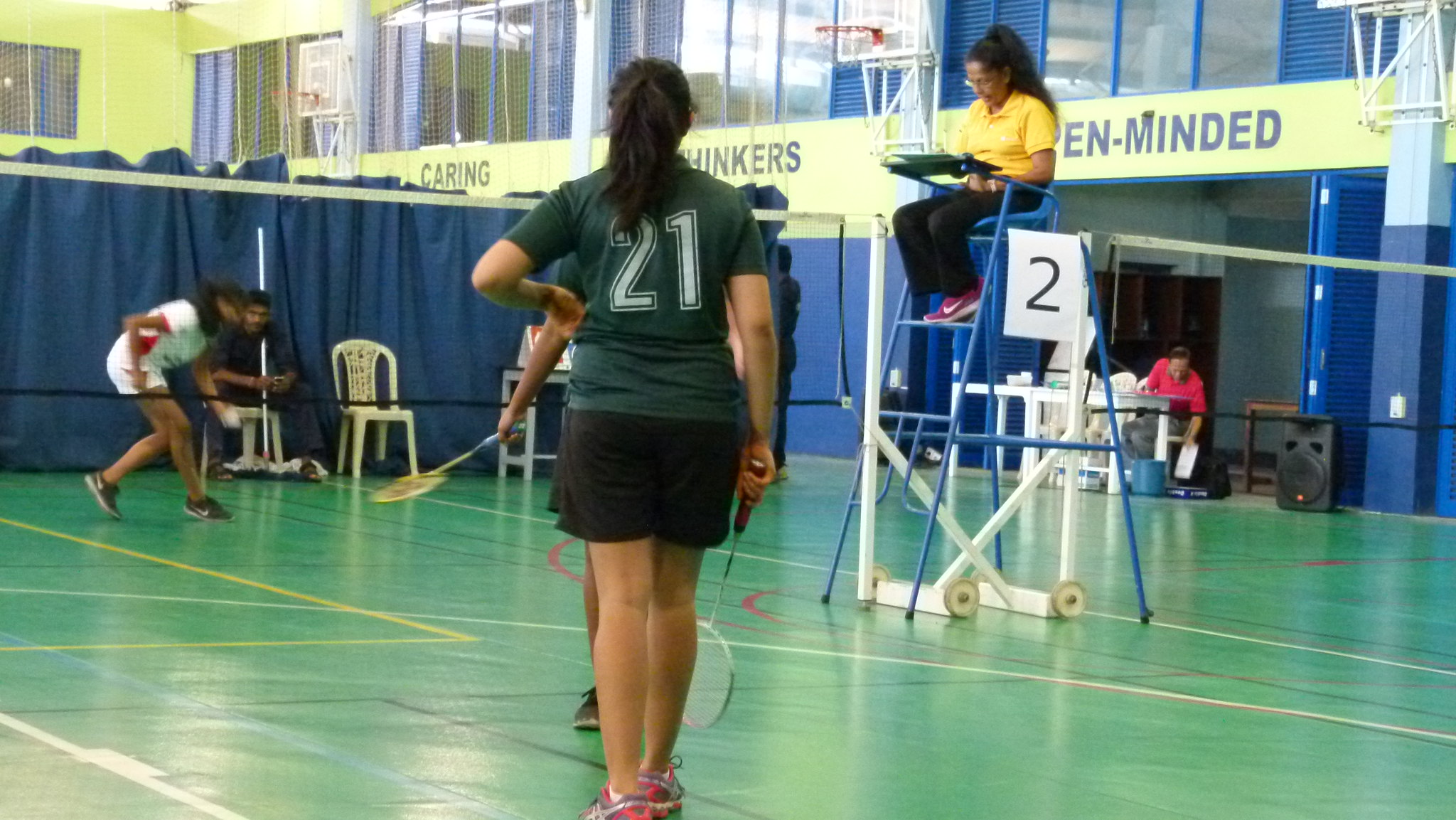In this detailed image of a badminton game taking place indoors, we see young female players in action on a vividly green court marked with various colored lines. The dominant figure in the foreground is a girl with dark hair tied in a ponytail, wearing a green short-sleeved team uniform with the number 21 on the back and dark shorts. She holds a badminton racket mid-play. Partially visible behind her is another player, identifiable by glimpses of her arm, racket, and leg. To the left, the opponents can be seen, preparing for their next move.

On the right side of the image, a yellow-shirted scorekeeper, identified by her position atop a tall blue chair, is observing the game. Her perch prominently displays a sign with the number two. Directly below this, a folded white paper is attached to the stand. Nearby, a blue curtain runs along the wall, contrasting against the gym's white upper walls with windows and text. In the background, a man can be seen watching the game, adding to the scene's dynamic atmosphere. The overall setting is brightly lit, showcasing the vibrant and engaging environment of the sports activity.